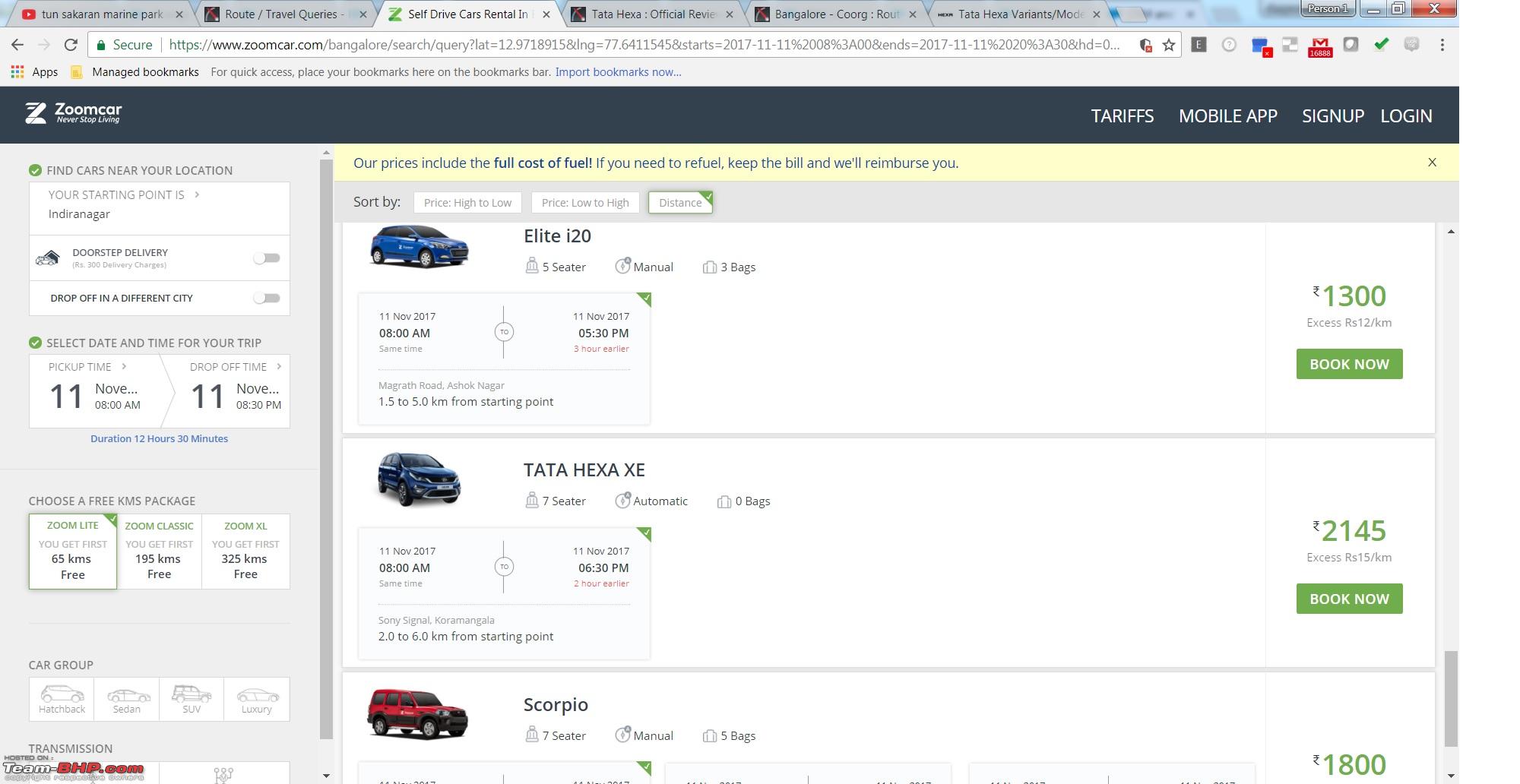A web browser is displayed with six tabs open. The first tab is a YouTube page titled "Tourist the Car and Marine Park." The second tab is labeled "Route Travel Queries," while the third one is for "Self-Drive Car Rentals." The fourth tab features a page titled "Tata Hexa Official Review," followed by a fifth tab labeled "Bangalore." The sixth and final tab is titled "Tata Hexa Variant."

Beneath the tab bar, a prominent section of the screen showcases a car rental service with the brand "Zoom Car." The slogan "Never Stop Living" is visible alongside options to sign up or log in through a mobile app. The service advertises that "Our prices include the full cost of fuel. If you need to refuel, keep the bill and we'll reimburse you." The screen also includes sorting options such as "Price High to Low," "Price Low to High," and "Distance."

A specific car listing is highlighted with a blue card that reads "Elite i20," describing it as a five-seater, manual transmission vehicle with the capacity for three bags. The excess charge is noted to be $1,300 and includes a mileage limit of 12 kilometers. A green "Book Now" button is prominently displayed under the listing.